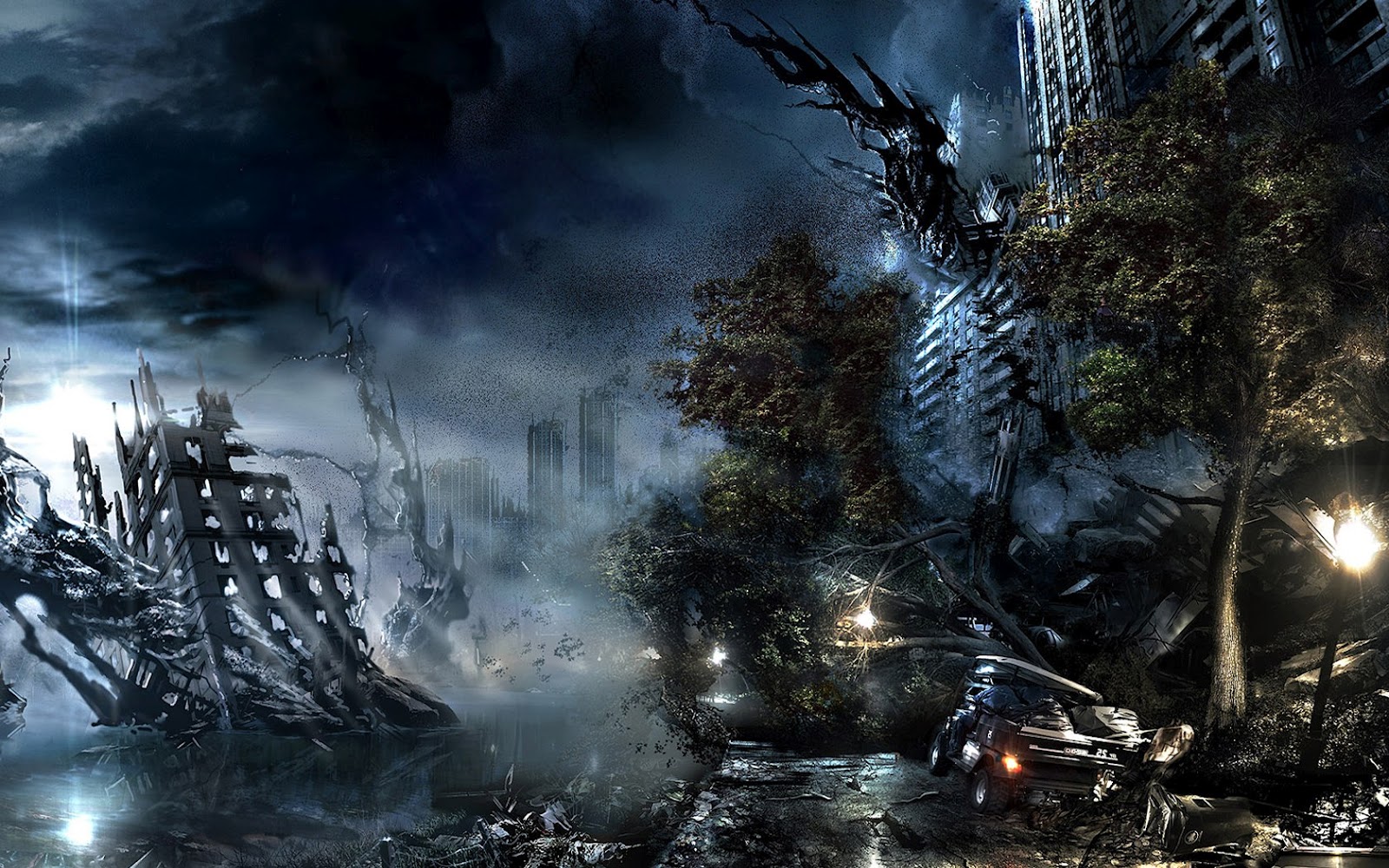The image depicts a cityscape that has been ravaged by a severe natural disaster or possibly a war. The scene is engulfed in a dark, cloudy sky with very little light penetrating through the gloom, creating a dreary and apocalyptic atmosphere. The destruction is evident with numerous buildings collapsing, including one prominently fallen over on the lower left corner. The night setting amplifies the devastation, with a windstorm adding to the chaos as trees are blown and fallen across the scene. A crushed car lies on the right side near a road, further emphasizing the catastrophe. There is a faint light source in the background, potentially hinting at a nuclear explosion or another violent event. Central and left middle parts of the image feature reflections of light on the ground, providing a stark contrast to the otherwise dark tones. Some skyscrapers in the middle of the image remain standing amid the extensive destruction, underscoring the severity of the disaster faced by this city.